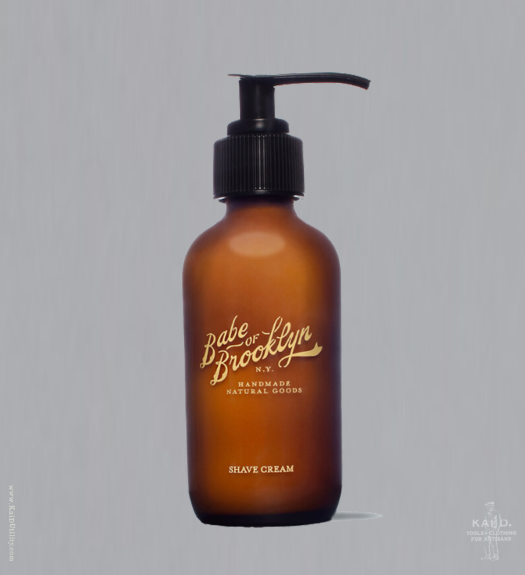The image features a bronze-colored bottle, possibly made of plastic or glass, with a black cap and pump dispenser oriented to the right side. The bottle prominently displays the brand name "Babe of Brooklyn" in yellow script text, followed by "New York" in capital printed letters. Below, "Handmade Natural Goods" and "Shave Cream" are printed in capital letters similar to "New York," with "Shave Cream" being slightly larger. The bottle is set against a plain gray background, giving it a floating appearance. In the bottom right-hand corner, there is a watermark that reads "KAUD, Tools and Clothing for Artisans," alongside a small figure of a man. Additionally, along the left side, a website URL, www.caldutilities.com, is visible. The clean and minimalist design suggests that the image might be part of a magazine advertisement.